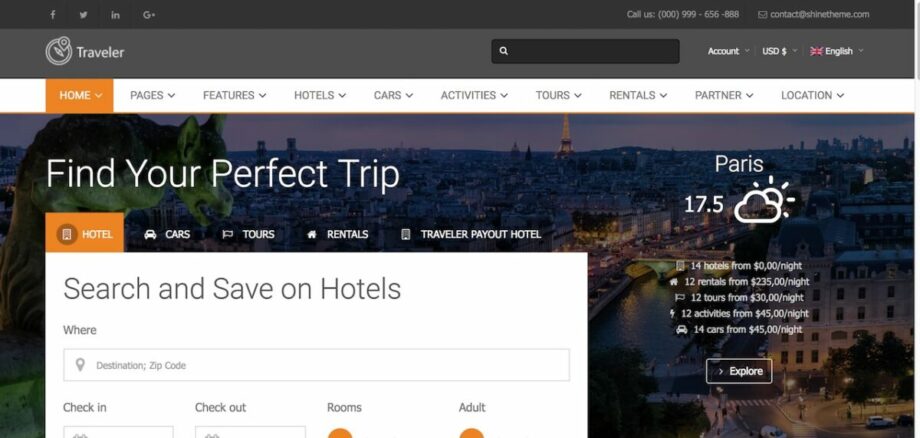The rectangular image, with its longer side extending horizontally, features a prominent black border at the top. Within this border are faint white inscriptions, including symbols for Facebook and Twitter, followed by "N" and "G+" on the left-hand side. On the right-hand side, there is a contact number with the text "Call us," and what appears to be an email address.

Beneath this black border is a lighter gray box that starts from the left with the word "traveler," next to a search box marked by a search icon. Further right, this section includes options for "Account," "USD," and "English," the last accompanied by a small British flag.

Immediately below this lighter gray box is another banner, which runs horizontally across the page and is white in color. On the top left of this banner, an orange box highlights the word "Home" in white letters. A drop-down menu accompanies "Home," as well as the subsequent tabs: Pages, Features, Hotels, Cars, Activities, Tours, Rentals, Partner, and Location, each of which also has a drop-down menu.

Moving to the main body of the image, bold text reads "Find your perfect trip." Below this heading, several tabs are displayed, with the "Hotel" tab selected and highlighted in orange with white text. The other tabs include Cars, Tours, Rentals, Travel, and Payout. Positioned below these tabs, a white box instructs users to "Search and save on hotels."